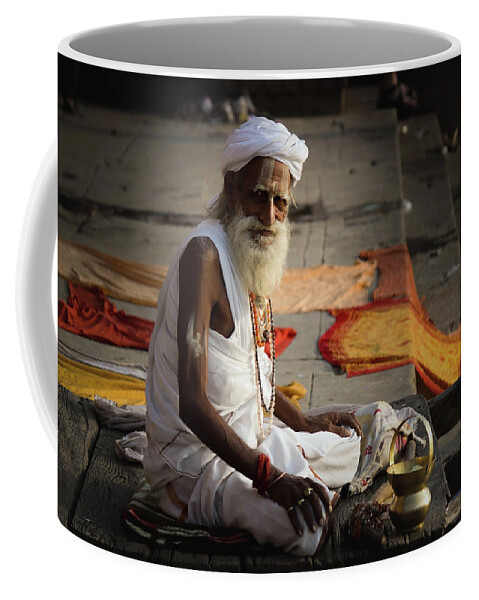This is a close-up image of a customized coffee mug, showcasing an intricate and evocative scene of an Indian man. The handle of the coffee mug is white, visible only slightly from the front view, allowing a peek into the white interior of the mug. Encircling the mug is a detailed picture that captures an older, very thin Indian man sitting on a carpet or rug laid out on a concrete floor, surrounded by a vibrant array of draped fabrics. Some fabrics are silky red or maroon, others are yellow with red borders, and further back are light orange fabrics.

The man, dressed entirely in white, including a white headdress or turban, white cut-off shirt, and white pants, is seated on the ground. He is adorned with rings on every finger, a gold bracelet on one wrist, and red fabric wrapped around his other wrist. Around his neck, he wears beads. He directs his gaze towards the camera, turning his head slightly to the side but keeping a direct and intense eye contact.

In front of him, resting on the ground, is a gold mortar and pestle, possibly used for some ritualistic or daily activity. The background reveals a cluttered scene with litter scattered across the concrete steps, adding to the narrative depth of the man's setting. The intricate details and rich colors depicted on the coffee mug capture a moment that hints at the man's cultural and personal story.